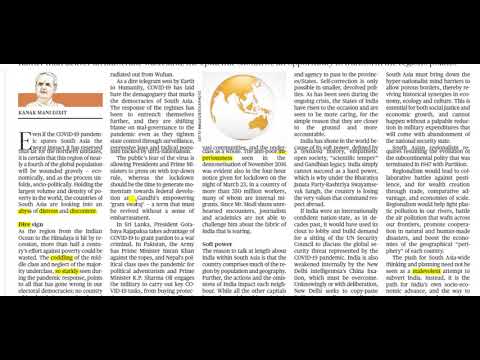The image appears to be a photograph of a newspaper article, organized into five columns of largely illegible text against a white background. Scattered throughout the text are sections highlighted in yellow. Dominating the center is a stylized globe, depicted in white with orangish landmasses outlining the continents. To the top left corner, an outlined drawing of a short-haired person—presumably a man—stands in front of an orange banner. Although the accompanying text is unclear, the visible portion suggests the start of a word with "K" or "M-A-K," possibly related to management.